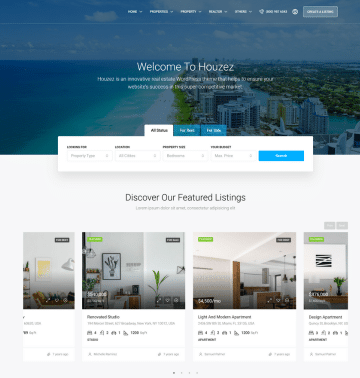The image depicts a webpage from a travel rental website called "Houzez" (spelled H-O-U-Z-E-Z). The top banner of the webpage features a picturesque beach scene with condos and apartments lining the shoreline, giving a serene and inviting impression. Prominent text in the banner reads "Welcome to Houses."

Above the banner, there is a navigation menu with five drop-down items, suggesting various categories or options for browsing the site. 

Below the banner, a section titled "Discover our Featured Listings" showcases various property listings. This section includes a horizontally scrolling carousel with images of different rental properties, each accompanied by key details such as the number of bedrooms, bathrooms, and the overall size of the property.